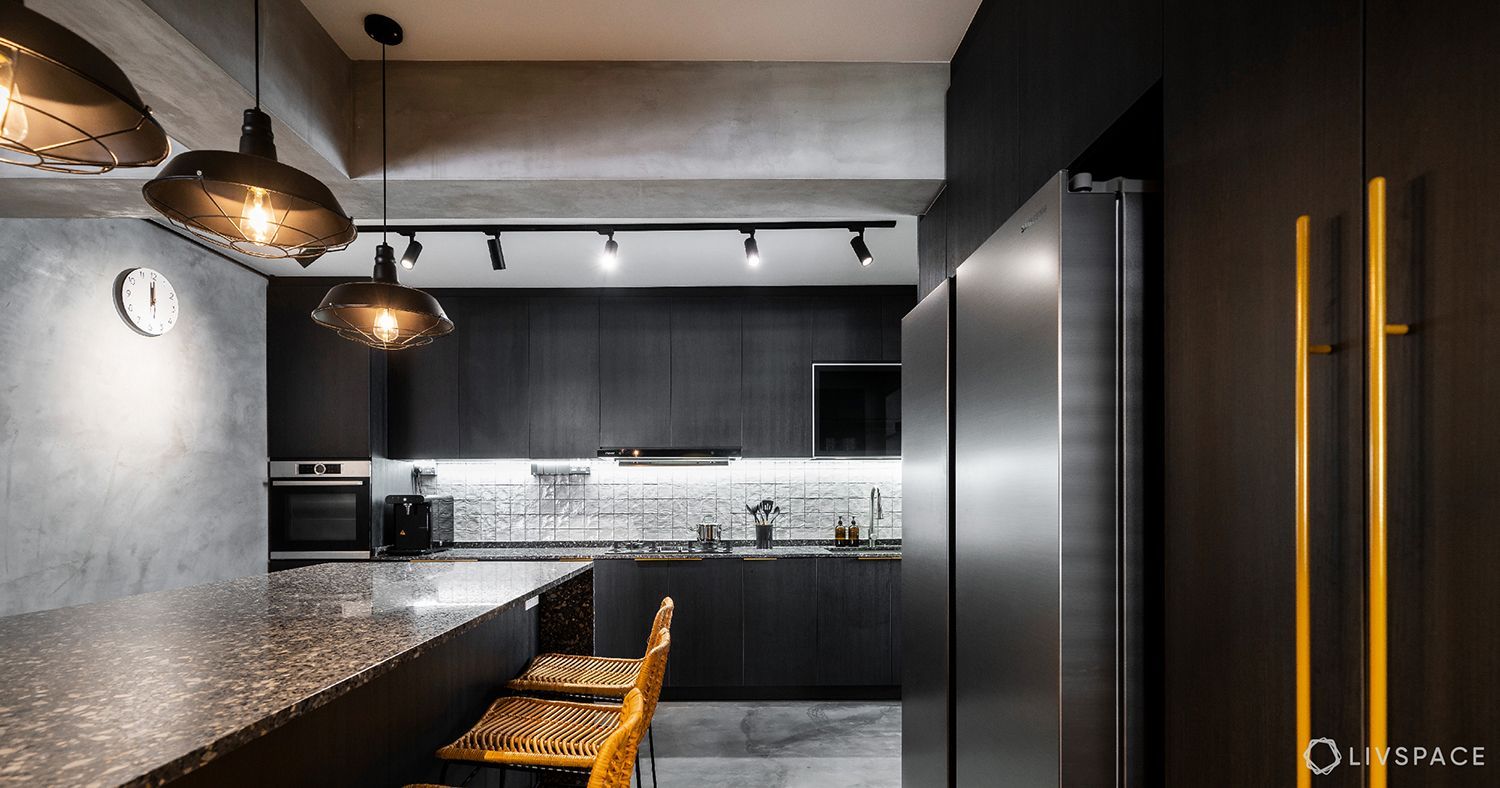This image showcases a sleek, contemporary kitchen featuring a prominent granite island equipped with two yellowish-golden chairs. Suspended above the island are three elegant light fixtures. To the left, there's a gray marble backsplash wall adorned with a white clock. Dark cabinets with large gold handles line the far wall, complementing a white tile backsplash. Integrated into this backdrop are various stainless steel appliances, including an oven, an air fryer, and a microwave situated above. On the right side stands a double-door stainless steel refrigerator without visible handles, suggesting a modern, handle-less design. The sink, complete with two soap dispensers filled with a brown liquid, is positioned below the cabinets, which are finished in gray. The bottom right-hand corner of the image features a small white symbol that reads "LIVE SPACE," indicating the possible branding or photographer's mark. Overall, the kitchen's design emphasizes a sleek, functional aesthetic with consistent gray tones and high-end materials.